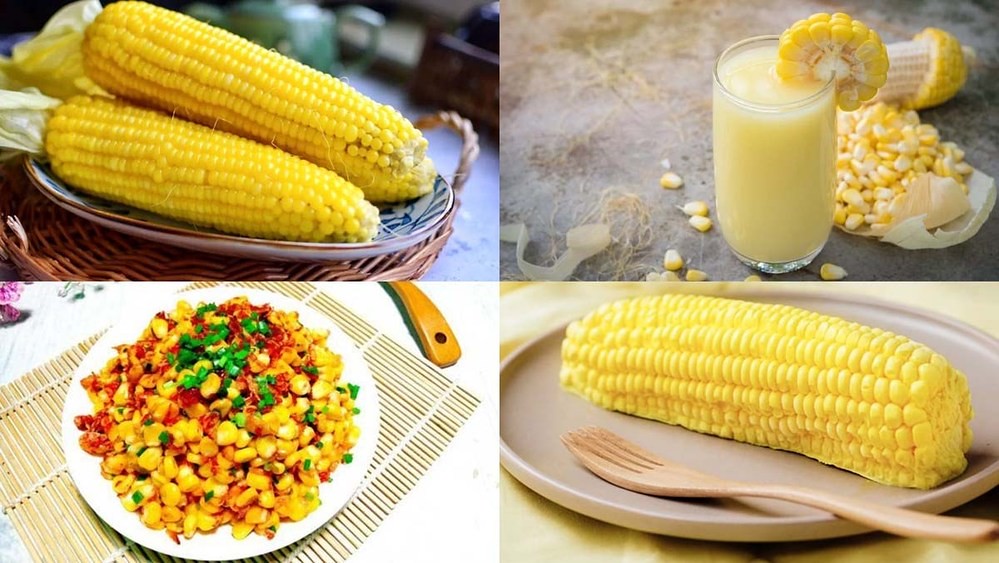This image features a collage of four distinct photographs showcasing various ways to use corn. In the top left, there are two bright yellow corns on the cob positioned on a white plate with a dark blue pattern and a golden rim, which is placed on a woven tray. A tea kettle and drawers are subtly visible in the background. The top right image displays a unique corn drink in a tall glass, light yellow in color, with a slice of corn on the cob decoratively perched on the rim, reminiscent of a cocktail garnish. In the background, there's a gray surface with both corn kernels and a shaved corn cob. The bottom left picture presents a meal featuring corn mixed with red and green ingredients, possibly bacon bits and herbs like coriander or parsley, served on a white plate atop a bamboo mat, with a wooden ladle partially visible. The bottom right shows a single corn on the cob, seemingly lathered in butter, on a light brown, flat plate accompanied by a brown fork, with a yellow cloth underneath.